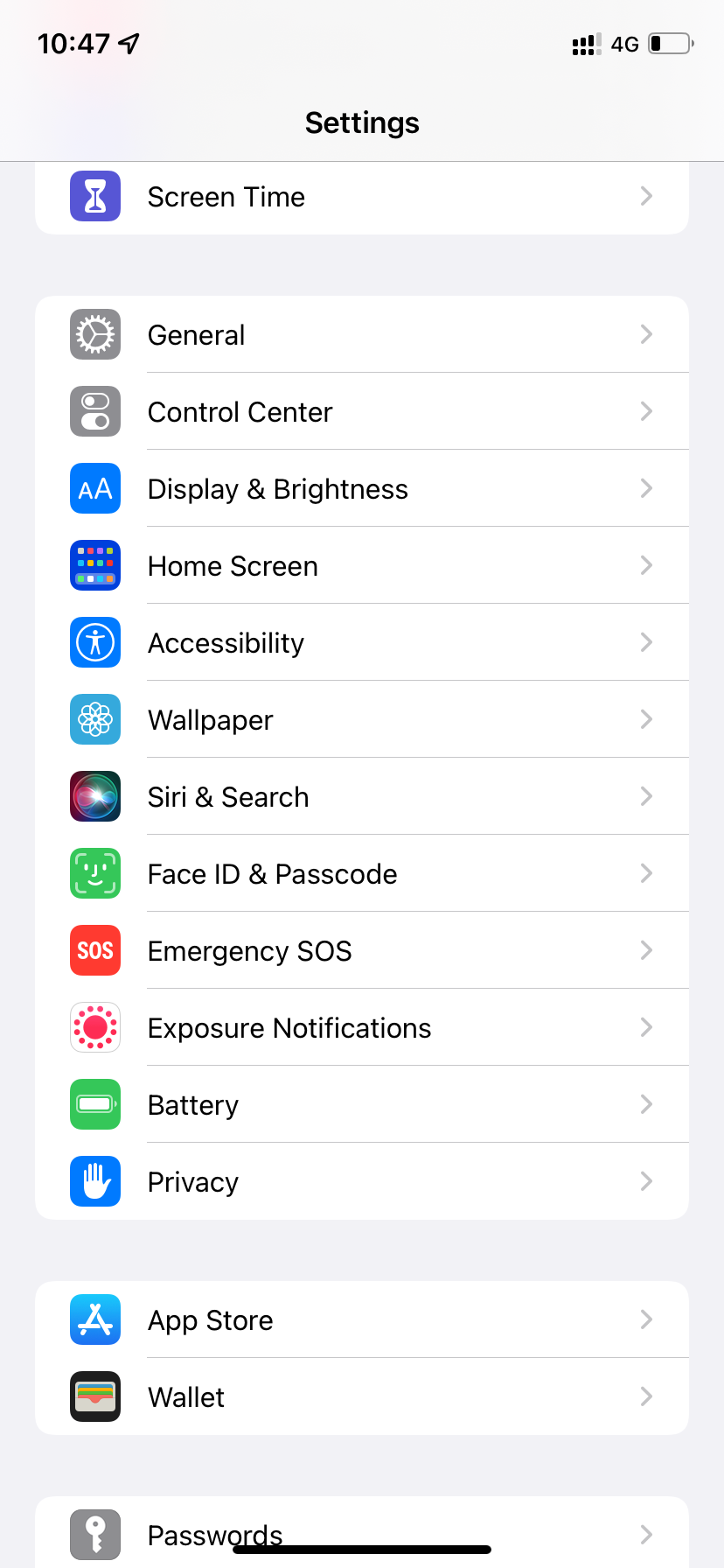The image shows a detailed screenshot of an iPhone's "Settings" menu taken at 10:47 AM in light mode, evident by the white background. Each category is accompanied by a distinct icon: 

- "Screen Time" appears at the top of the list without an accompanying icon.
- "General" is represented by a gear icon.
- "Control Center" and "Display & Brightness" are prominently displayed.
- "Home Screen," "Accessibility" (illustrated with a Vitruvian man icon), and "Wallpaper" follow.
- "Siri & Search," "Face ID & Passcode," and "Emergency SOS" (marked by a red box with "SOS").
- Further down, "Exposure Notifications," "Notifications," "Battery" (currently at 20%), and "Privacy" (featuring a hand icon) are visible.
- The "App Store" is listed as well, with the scrollable menu suggesting more options below.

The battery level is at a critical 20%, and the network reception shows 3-4 bars, indicating a decent connection. The layout allows for scrolling both up and down to access additional settings not fully visible in the screenshot.